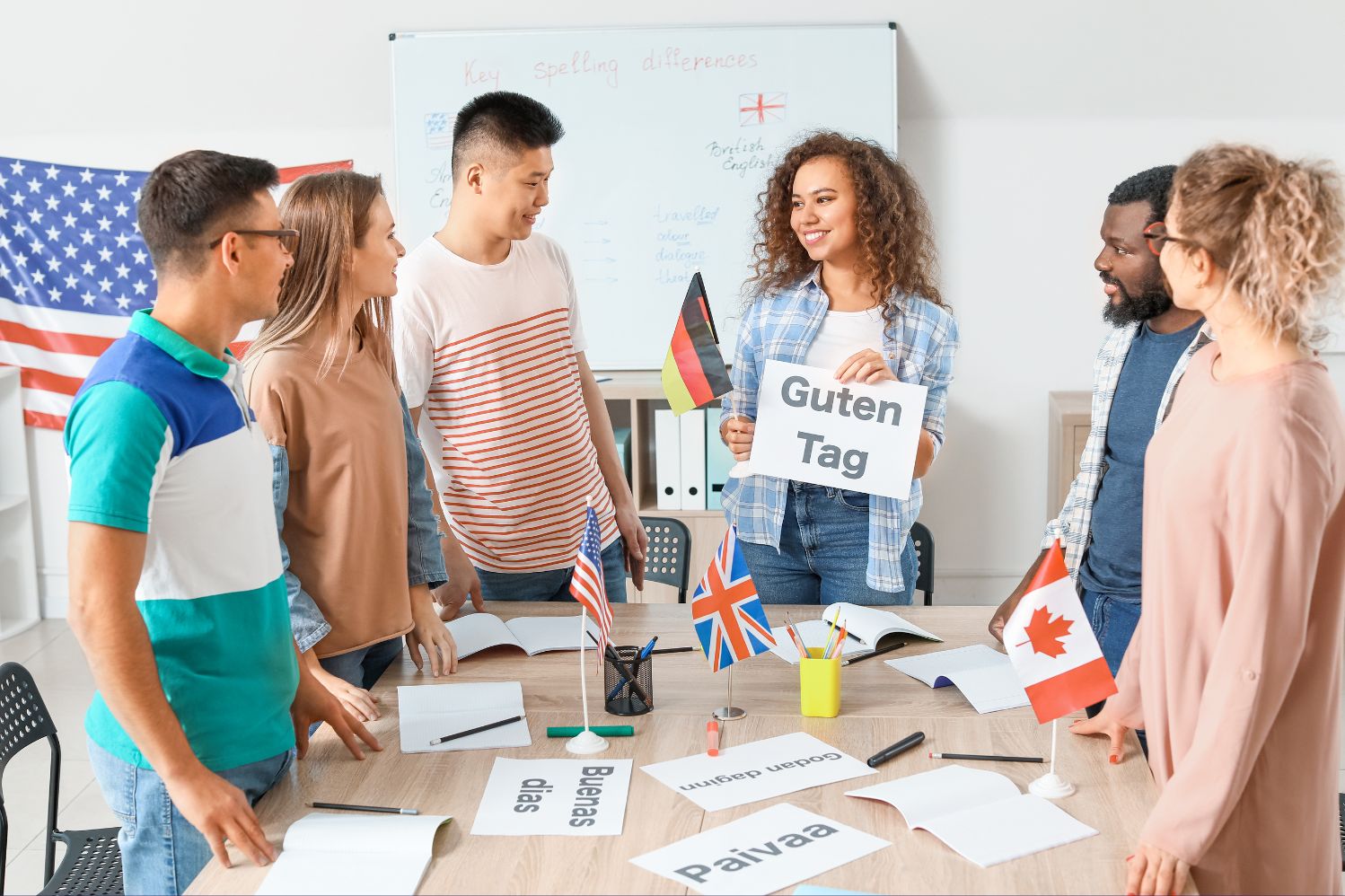In a well-lit room with a white wall and beige tiled floor, six people of varying races and genders stand around a rectangular table, engaging in a lively discussion. Dominating the left side of the wall is a vibrant American flag, complemented by a whiteboard positioned centrally, which features the red-ink heading "Key Spelling Differences" and hastily drawn illustrations of the American and British flags labeled "American English" and "British English," respectively. On the table, an array of flags — the American, Union Jack, and Canadian — are spread out with accompanying papers inscribed with greetings in different languages, such as "Buenos Dias," "Golden Dagen," and "Paiva."

To the left, a man with short brown hair and glasses, wearing a white, aqua blue, and dark blue striped polo shirt, stands beside a woman in a light brown shirt with long brown hair. At the far end of the table, a man in blue jeans and a white t-shirt with thin red stripes and short black hair is present. Central to the group is a woman with long brown curly hair, smiling broadly, dressed in blue jeans, a white shirt, and a blue and white striped plaid shirt. She holds a sign reading "Guten Tag" in black text and a German flag in her right hand, drawing the group's attention. To the right, a bearded man in blue jeans, a blue t-shirt, and a blue and white striped flannel shirt stands beside a woman with bleach blonde curly hair, wearing a pinkish-brown long-sleeve shirt and red-rimmed glasses. The image captures a moment of shared cultural learning and interaction.